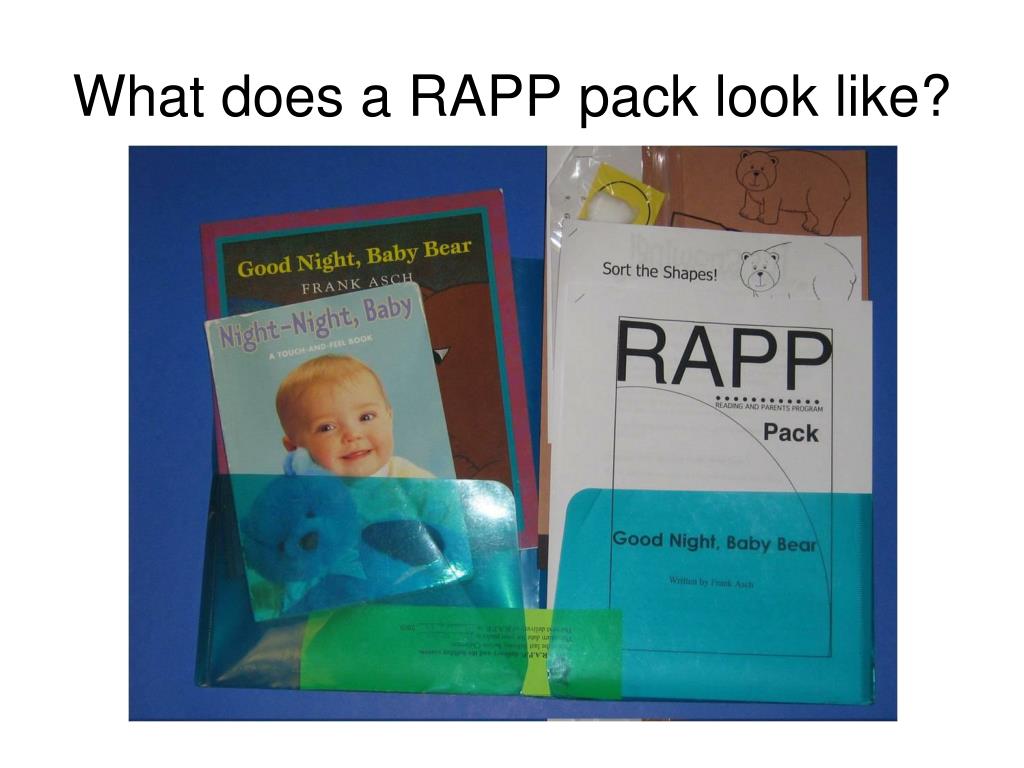The image titled "What does a RAPP pack look like?" displays an open blue plastic folder against a brighter blue background. The folder has two transparent pockets that reveal its contents. In the right pocket, there are two books. The book at the front, titled "Night Night Baby," has a light blue cover featuring a baby holding a blue teddy bear. Behind it is another book titled "Good Night Baby Bear" by Frank Ash, identifiable by its magenta border and a sketch of a bear on the cover. Additionally, there's a RAPP pack, which stands for Reading and Parents Program, also labeled "Good Night Baby Bear," visible through the pocket. The contents suggest these materials are likely sent home for reading activities.